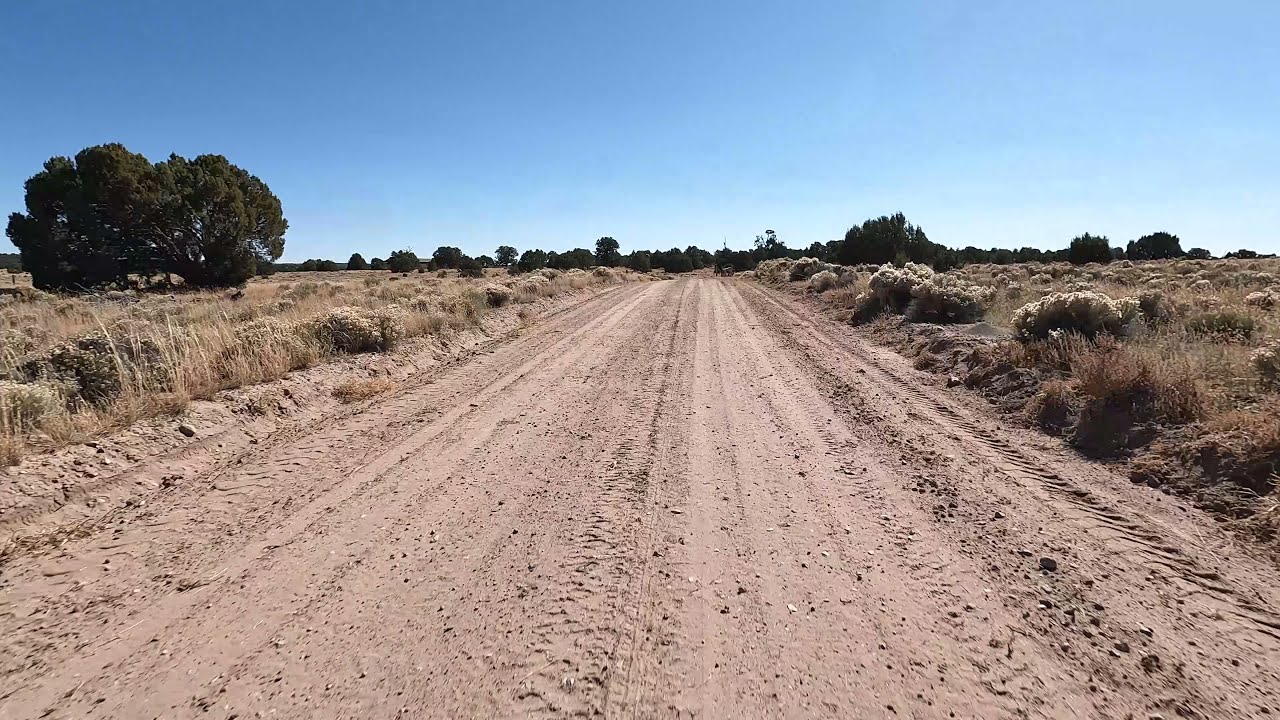This horizontally aligned rectangular image captures a seemingly endless dirt road stretching through a rural area under a clear, bright, blue sky. The road, flanked by dry, tall brown grass interspersed with sporadic bushes, is wide enough to resemble a two-lane pathway, marked by prominent tire tracks suggesting it is frequently used by large vehicles for off-roading. The terrain is flat with numerous rocks and sandy patches, showing signs of ruggedness and wear. On the left side, two decent-sized green trees stand side by side in the upper corner, with more scattered trees visible further in the background and on the right side. The road, devoid of any people, extends straight into the horizon with no curves, lined by weeds protruding from the ground. A tiny vehicle can be glimpsed in the distance on the right side of the road, enhancing the sense of scale and solitary expanse. The composition is simple and serene, dominated by the natural earthy elements and vast open sky.